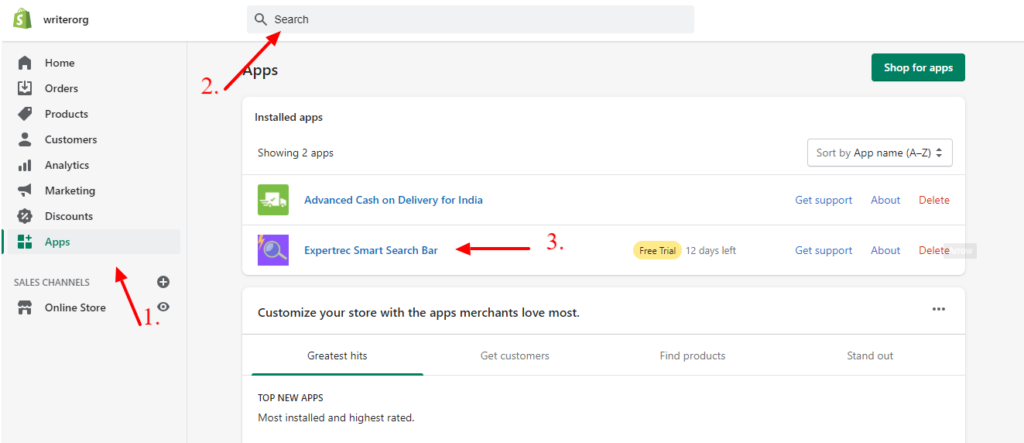### Detailed Description of the Screenshot:

The image appears to be a screenshot of a search interface on a website identified as Writer.org, with visual elements and several interactive components.

- **Top Left Corner**: The site is branded with the name "Writer.org."
- **Left Sidebar**: The sidebar features a vertical menu with several widgets. The items listed include:
  - **Home**
  - **Orders**
  - **Products**
  - **Customers**
  - **Analytics**
  - **Marketing**
  - **Discounts**
  - **Apps**: This is highlighted with teal text, a light gray highlight bar, and a vertical teal indicator on the left.

- **Iconography**: 
  - At the top of the sidebar, there is a green icon that resembles a money bag with a dollar symbol ($) on it.

- **Background**: The general background of the site is a light gray color. 
- **Main Content Area**:
  - **Central Part**: The central part of the screen is primarily white.
  - **Search Functionality**:
    - There's a search bar located to the right side of the Writer.org logo.
    - Below the search bar, a teal button with white text reads "Shop for Apps."
    - Below this button, the text "Installed Apps" is visible.
  - **Sales Channels**:
    - An arrow points upwards from the "Sales Channels" section. This indicates that users can manage various sales channels, with "Online Store" being one option listed in gray text.
  - **App Listings**:
    - **Sorting Options**:
      - The interface allows sorting by app name (A-Z) via a dropdown menu.
    - **App Entry #1**:
      - **Icon**: Green icon on the left.
      - **Title**: A blue link labeled "Advanced Cash on Delivery" (specific to the Indian market).
      - **Actions**: On the right are three clickable options - "Get Support," "About" (both in blue), and "Delete" (in red).
    - **App Entry #2**:
      - **Icon**: Purple icon on the left.
      - **Title**: "Expert Text Smart Search Bar."
      - **Free Trial Info**: Indicates there are 12 days left on a free trial.
      - **Actions**: Similar options - "Get Support," "About," and "Delete."
    - **Other Sections**:
      - "Customize Your Store"
      - "Apps Merchants Love Most"
      - "Greatest Hits"
      - "Top New Apps"
      - "More Installed"
      - "Highest Rated"

Overall, the screenshot presents an organized, user-centric dashboard that allows easy navigation and management of various applications, along with a robust search functionality for app discovery and sorting options.